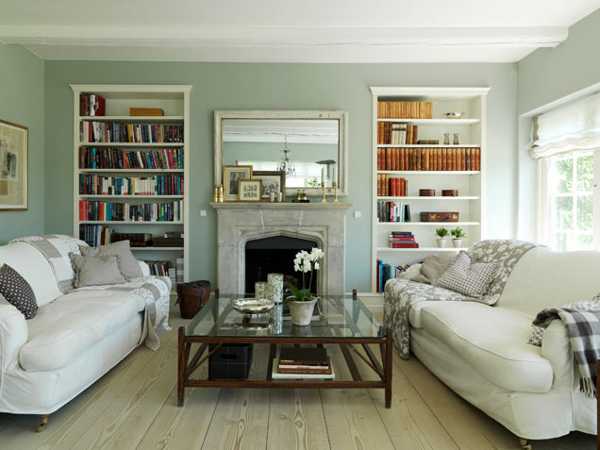The photograph features a tastefully decorated living room with a sophisticated ambiance. The perspective looks towards the back wall, which is highlighted by a centrally placed unlit fireplace. Above the fireplace hangs a rectangular framed mirror, flanked by built-in white bookcases on either side. The left bookcase is densely packed with books and possibly DVDs, whereas the right contains a set of encyclopedias along with various decorative items, including plants, chests, and candles. 

In front of each bookcase extends a pristine white couch, adorned with an assortment of light gray, white, and black blankets and pillows. These couches lead towards the viewer, framing a glass coffee table in the center, which features wooden legs and an underframe. The table is decorated with a plant, a couple of candles, and a bowl.

The room's color palette consists predominantly of light tones, with seafoam green walls providing a subtle backdrop that complements the white ceiling and white painted beam running across it. The space is further brightened by natural sunlight streaming through an open window on the right wall behind the sofa. The floor is a warm hardwood, adding a touch of natural texture to the setting. A painting is visible on the left wall above the couch, contributing to the room’s polished and tranquil atmosphere.